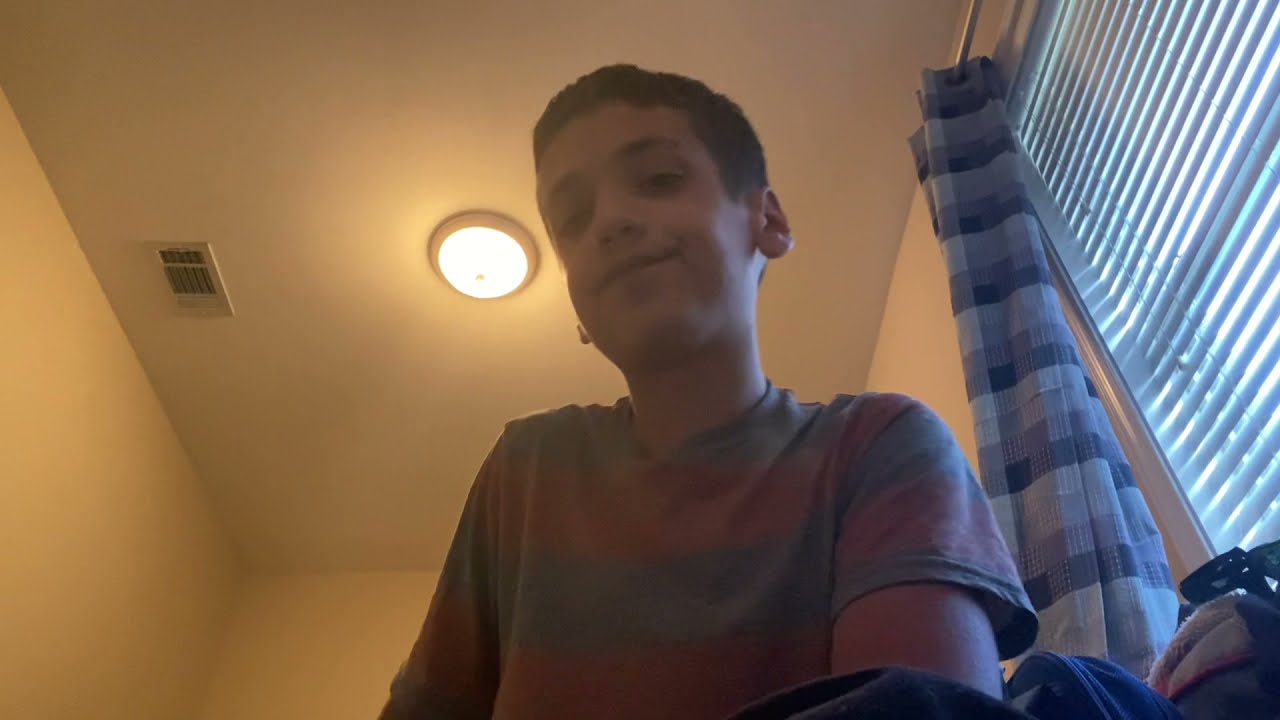The image is a photograph of a young Caucasian boy, likely between the ages of 10 to 15, taken from an upward angle as if the camera is placed on the floor. The boy has short brown hair and light skin, and he’s looking down at the camera with a closed-mouth smirk, giving off a playful, slightly amused expression. He’s wearing a short-sleeved t-shirt featuring blue and red stripes. The lighting in the room is a warm yellowy-orange, casting a shadowy hue over the scene. Behind him, you can see a ceiling with a round light fixture casting a soft glow, and a white vent nearby. To the right of the boy, there is a window with partially closed white horizontal blinds and blue checkered curtains.